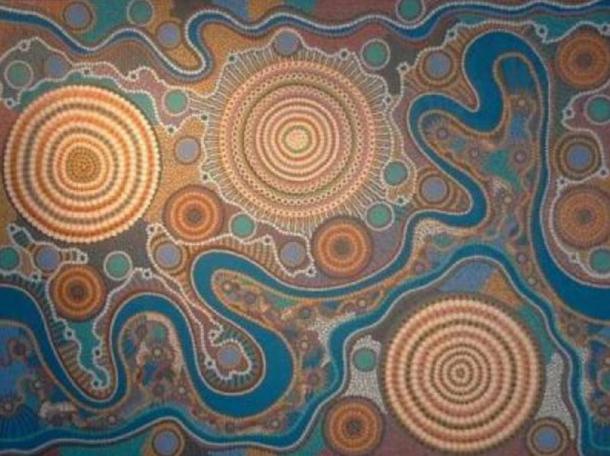The image is a rectangular piece of abstract, psychedelic artwork that takes up the entirety of the frame, lacking any discernible text or identifiable objects. Dominated by vibrant colors including shades of orange, red, yellow, blue, turquoise, black, white, purple, pink, and various greens, the composition features three prominent, non-symmetrically placed circles. Two of these major circles are positioned near the top left, while the third is closer to the bottom right. Interwoven through these larger circles is a snaking green line reminiscent of a river seen from an aerial perspective. Additionally, there are about five smaller circles dispersed throughout the image, each containing intricate concentric patterns in hues of gray, orange, tan, and other vivid colors. The entire artwork gives off a trippy, mosaic-like appearance, suggesting it could be a fabric design, tapestry, or floor mat viewed up close. The overall aesthetic is chaotic yet cohesive, with its flowing lines and vibrant, multi-colored blotches creating a mesmerizing and immersive visual experience.